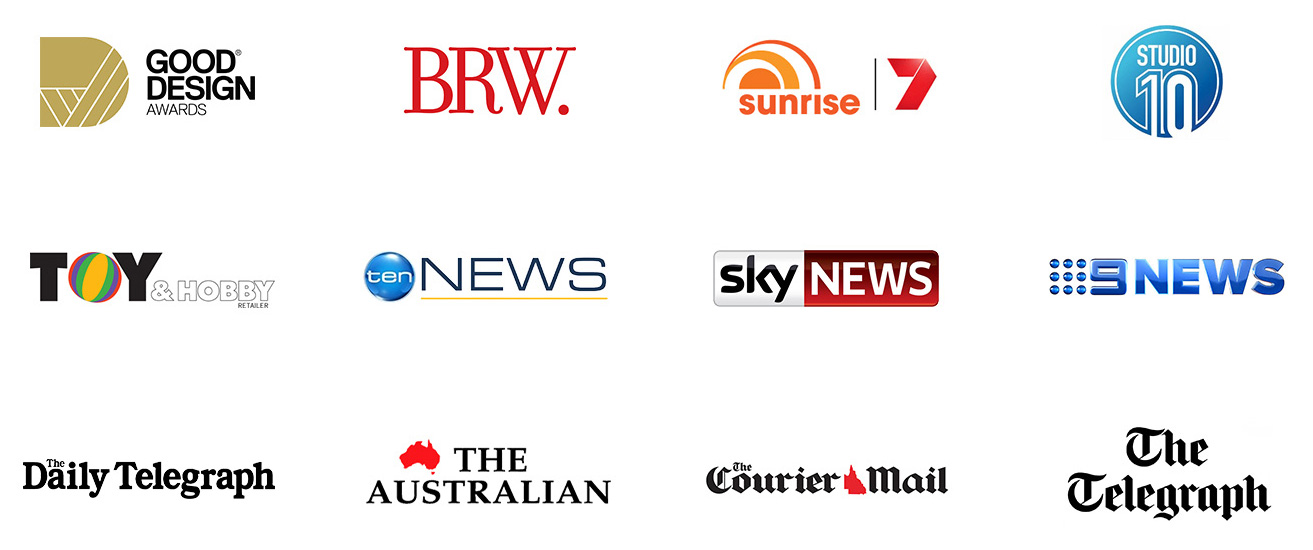The image is a screenshot taken from a laptop, showcasing an array of logos against a pristine white background. The logos are systematically arranged in three rows and four columns. 

In the upper left-hand corner, the first logo belongs to the Good Design Awards, followed by the BRW logo characterized by its distinctive red period. Next in line is the Sunrise 7 logo, which also features the color red. Completing the top row is the Studio 10 logo, distinguished by its aqua and digital-neon type styling.

The middle row begins with the Toy and Hobby logo, where the "O" resembles a rainbow-colored beach ball. This is followed by the 10 News, Sky News, and 9 News logos. Notably, the Sky News logo incorporates shades of red.

The bottom row starts with the Daily Telegraph logo on the left. Adjacent to it are the Australian logo, which includes a red image of Australia, and the Courier-Mail logo. Lastly, the bottom right-hand corner features the Telegraph logo. Between the Australian and Courier-Mail logos, there is a tiny red image.

Overall, the image showcases a diverse collection of logos, each with unique design elements and colors, effectively highlighting their brand identities.